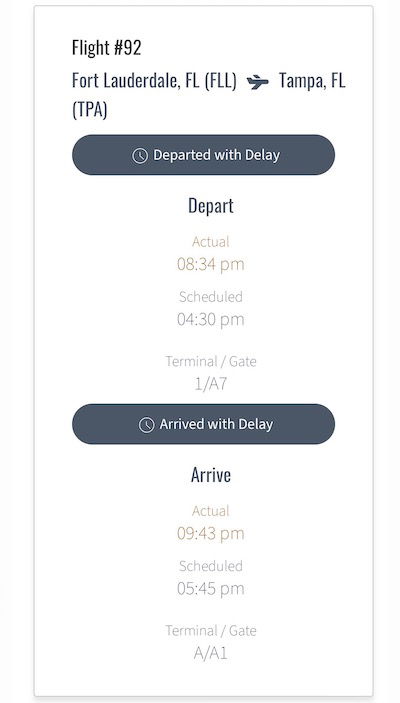Screenshot of a flight itinerary detailing a flight from Fort Lauderdale (FLL) to Tampa, Florida (TPA). The flight, labeled as Flight Number 92, shows important timetable information in black text. The itinerary indicates a departure with a delay: originally scheduled for 4:30 p.m., the actual departure time was 6:34 p.m. from Terminal Gate 187. The arrival was also delayed; the flight reached Tampa at 9:43 p.m., instead of the scheduled arrival time of 5:45 p.m., with Terminal and Gate A1 being notably indicated. The delays significantly impacted the travel time.